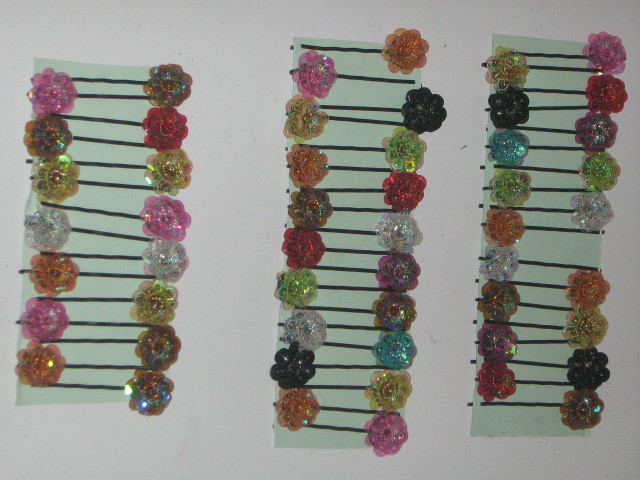The image showcases a hard, pale off-white or grayish surface adorned with three vertically arranged strips of cardboard, each harboring an array of bobby pins or hairpins. These strips run the entire length of the photo: one on the left, one in the center, and one on the right. The pins are attached to the cardboard backings, with the cardboard designed to accommodate each pin's arrangement. Each set features at least 10 to 11 pins, though some strips hold fewer.

The pins themselves are embellished with brightly colored, ornamental plastic flowers at their ends, displaying a variety of hues such as pink, yellow, orange, black, red, and dark purple. The flowers are somewhat translucent with a glittery interior, adding a touch of iridescence as light reflects off them. The flowers alternate in their attachment positions from the right side to the left side down the length of the strips. The overall presentation is both colorful and neat, with the flowers arranged in a way that suggests they are designed to appeal to a younger audience.